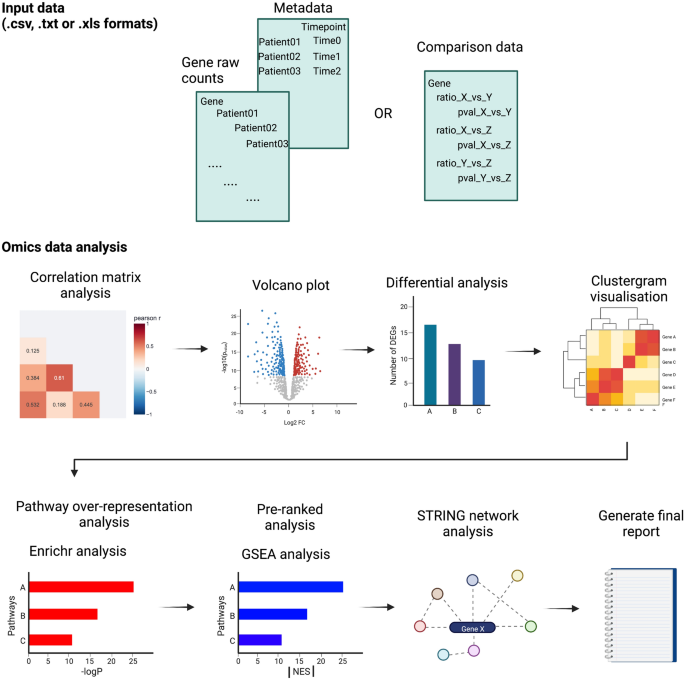The image is a detailed diagram elucidating the process of compiling and analyzing data to generate a final report, specifically in a medical context. The diagram is set against a white background and begins at the top with the title "Input Data," referencing formats like CSV, text, or XLS. Below this, three green rectangles signify the various types of input data: gene raw counts, metadata, and comparison data.

The middle section of the diagram is dedicated to "Omics Data Analysis," featuring four distinct types of data analysis techniques: 
1. Correlation Matrix Analysis, represented by a bar graph;
2. Volcano Plot Differential Analysis, depicted as a scatter plot on an X, Y axis;
3. A series of blocks with a gradient blur representing Differential Analysis;
4. Cluster Gram Visualization indicating clustered data.

An arrow from the Omics Data Analysis section points downward to another set of analyses, categorized into:
1. Pathway Over-Representation Analysis;
2. Enrichment Analysis (with a misinterpreted term "Enrique" corrected);
3. Pre-ranked Analysis using GSEA (Gene Set Enrichment Analysis);
4. String Network Analysis.

Finally, this sequence culminates in a section titled "Generate Final Report," marked by a final arrow pointing to a notebook icon. This final area includes colored vertical bar graphs (one red, one blue) and a network of circles connected by lines and dashed lines, symbolizing integrated data ready for report generation. The overall flow delineates how initial data inputs are systematically analyzed through various methods to produce a comprehensive final report.